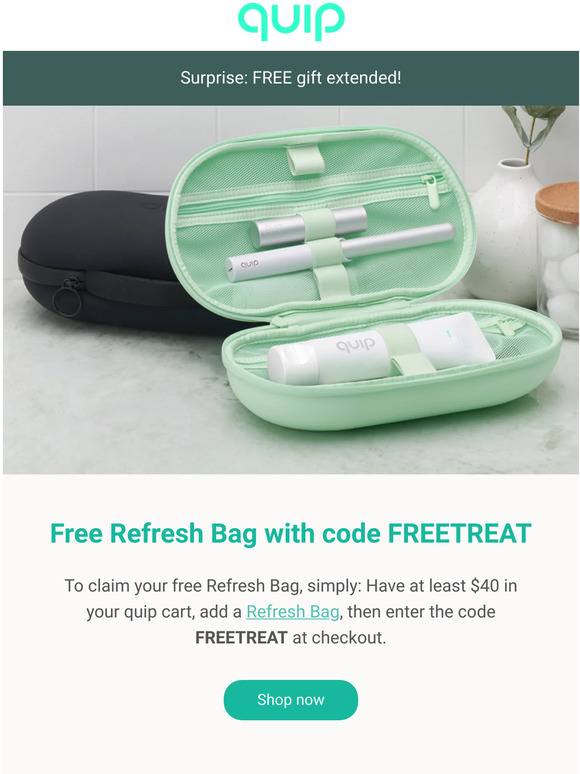A delightful surprise awaits! The image features a green zip-open pouch leaning against a sleek black pouch. Inside the green pouch, two silver tubes and a white squeeze tube bottle are perfectly nestled. To the right, there's a charming plant in a glass jar, and nearby, a jar with a brown lid filled with cotton balls. The scene is set against a white tile wall and a plush, furry floor. Don't miss out on this free refresh bag! To claim yours, simply have at least $40 in your cart, add the refresh bag to your order, and enter the code 'FREETREAT' at checkout. Shop now to get your free gift!